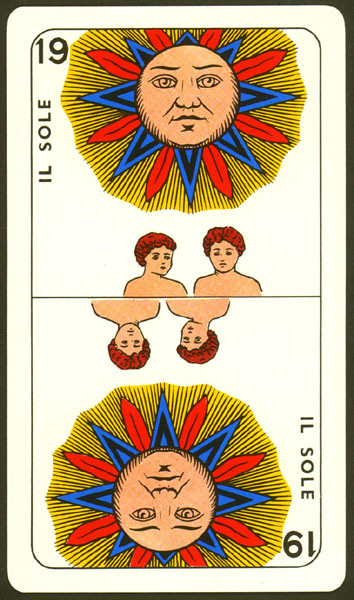This is an image of a tarot card titled "Ill Sole," representing the 19th card in the deck. The card features a central illustration of a face surrounded by petal-like sunbeams. These "sunbeams" deviate from the traditional yellow, instead, they are rendered in striking shades of red and blue. This face is encircled by an abstract yellow circle marked with small black striations that mimic the rays of the sun.

Beneath and above this central motif, two line-drawn human figures appear, depicted from the chest up with curly red hair and tan complexions. These figures are mirrored vertically, with one set right-side up and the other set upside-down at the bottom of the card, emphasizing the theme of duality. 

A thick black border frames the entire illustration, and a thin black line outlines the section with the image. Another thin black line bisects the card horizontally, accentuating the mirror imagery.

The card is labeled "Ill Sole" in all capital letters, with "I-L" as one word and "S-O-L-E" as another. The number 19 appears in the upper right-hand corner, with its mirrored counterpart in the lower left-hand corner, aligning with the mirror image theme. This distinctive and detailed card likely represents "The Sun" in the tarot deck, albeit with unique artistic interpretations.